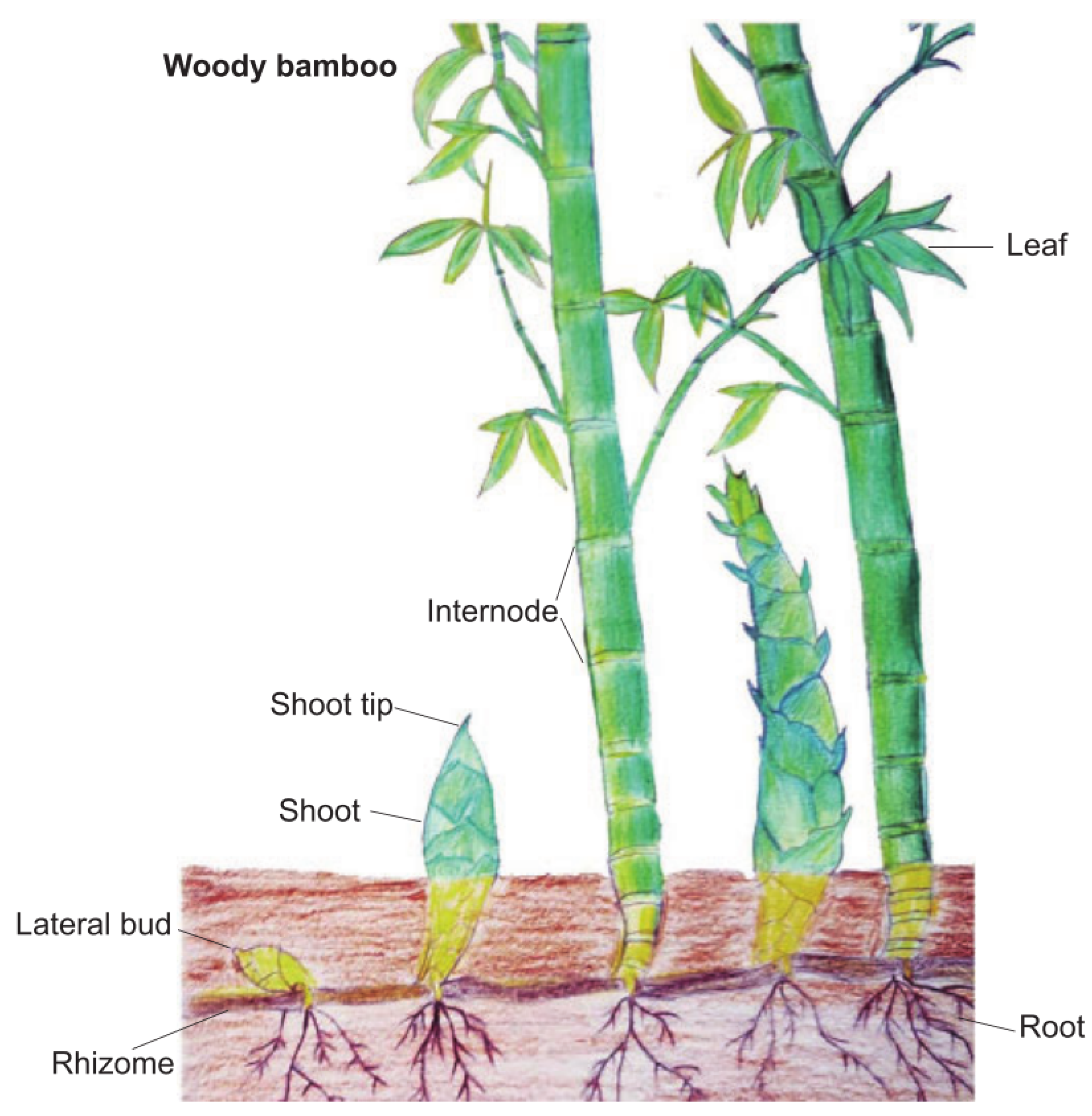This illustrated image vividly showcases the colorful and intricate growth stages of the woody bamboo plant. At the bottom, a layered representation of the ground is depicted with a blend of browns, mimicking the texture achieved with pencils and paint. Starting from the far left, the bamboo's growth is illustrated sequentially. It begins with a seed and shows its journey to becoming a full-grown bamboo, moving from left to right.

Annotations in black print clearly label each part of the bamboo at its various stages. On the leftmost part, the underground seedling is marked as "Rhizome lateral bud." As the bamboo grows, it transforms into a shoot that sprouts upward, identified as the "shoot tip." Progressing further, a labeled "internode" illustrates a larger bamboo segment. Finally, the diagram points to the "leaf" at the top of a mature bamboo stalk.

At the bottom right, the word "root" is labeled, pointing to the intricate underground root system that sustains the bamboo. The detailed depiction and precise labels make this illustration an informative guide to understanding the development of the bamboo plant from seed to maturity.